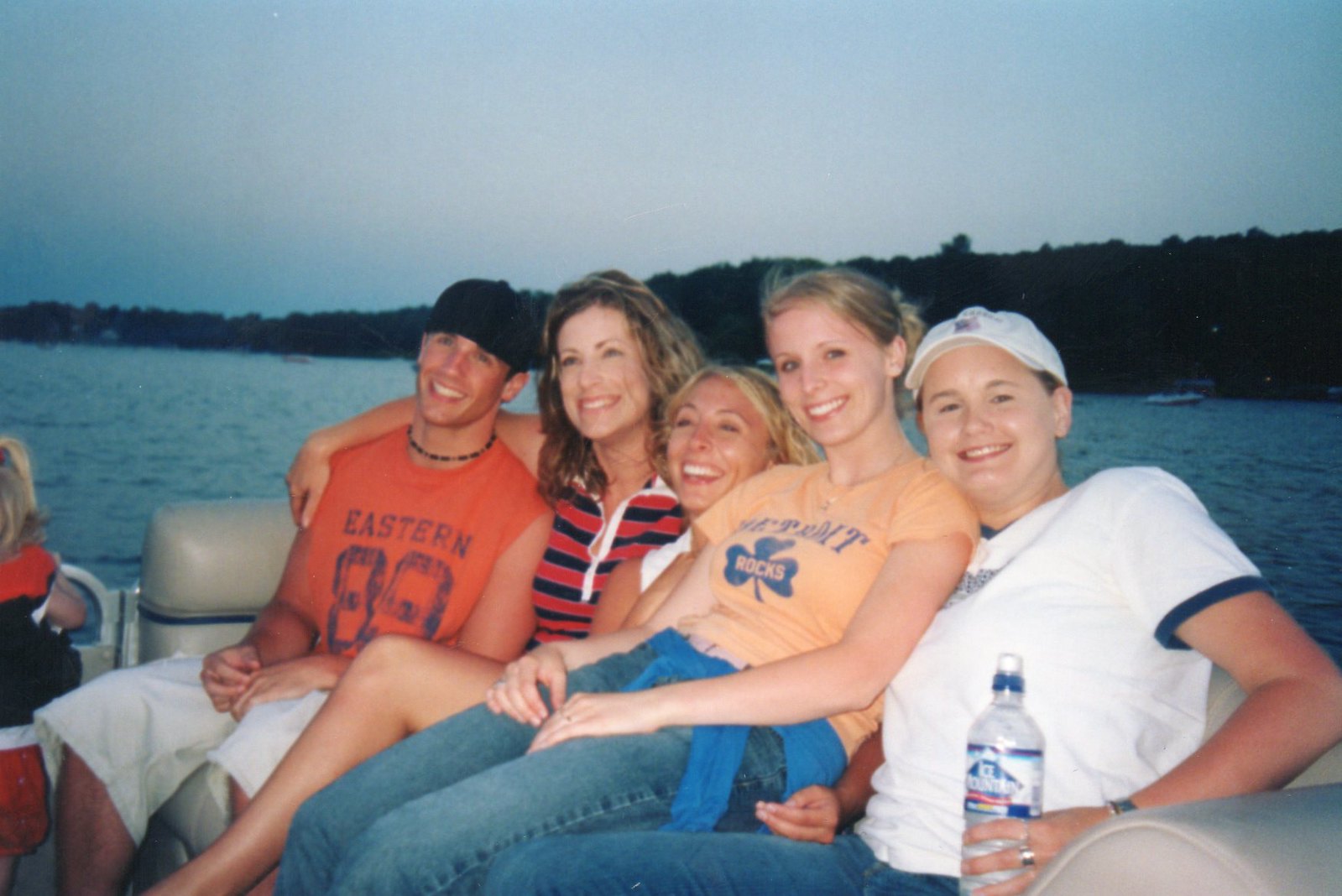In this vintage photograph, a group of five friends is captured enjoying a late afternoon on a boat, perhaps a small charter or tourist boat. The boat features grayish-white leather seats arranged like a long couch, where the group is lounging and posing for the photo. To the left of the frame sits a young man in his 20s, while the four women, ranging from late teens to their 20s, take up the remaining space on the couch. 

The three women in the middle all have blonde hair; one, who looks older and might be a mother, has long blonde hair and is wearing a red and blue striped shirt with her arm around the young man. Another has her hair tied back in a ponytail and is dressed in a yellow shirt. The woman on the far right is in a white T-shirt and a white baseball cap. The scene, set during the transition from day to evening, is illuminated by the dimming light, suggesting either late summer or early fall. 

The serene background showcases a large body of water, likely a lake or a wide river, bordered by mountains and darkened trees, adding to the tranquil and nostalgic atmosphere of the photo.